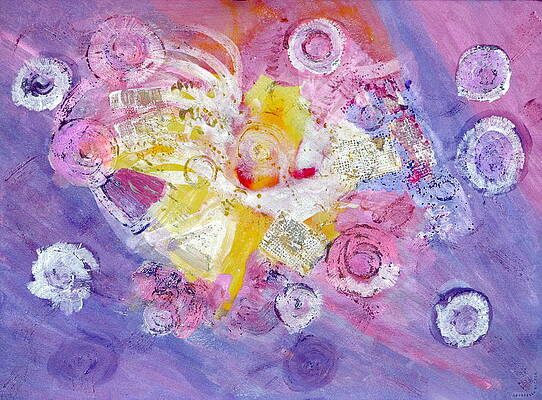The image is a scan of an abstract art piece with a predominantly purple and pink background. The corners are varying shades of purple, with the top right corner being a lighter lavender. The central focus of the painting features a complex and textured assembly of colors, including white, yellow, orange, and red, with some hints of blue brushstrokes. There are distinctive circular shapes resembling sushi slices scattered throughout the piece. These circular forms, mostly white with splashes of purple, pink, and lavender, surround a central vibrant spot that includes a mix of white, yellow, orange, and red hues. The entire composition is framed with the camera pointed directly at the surface, emphasizing the tactile quality of the textured circles against the richly colored background.